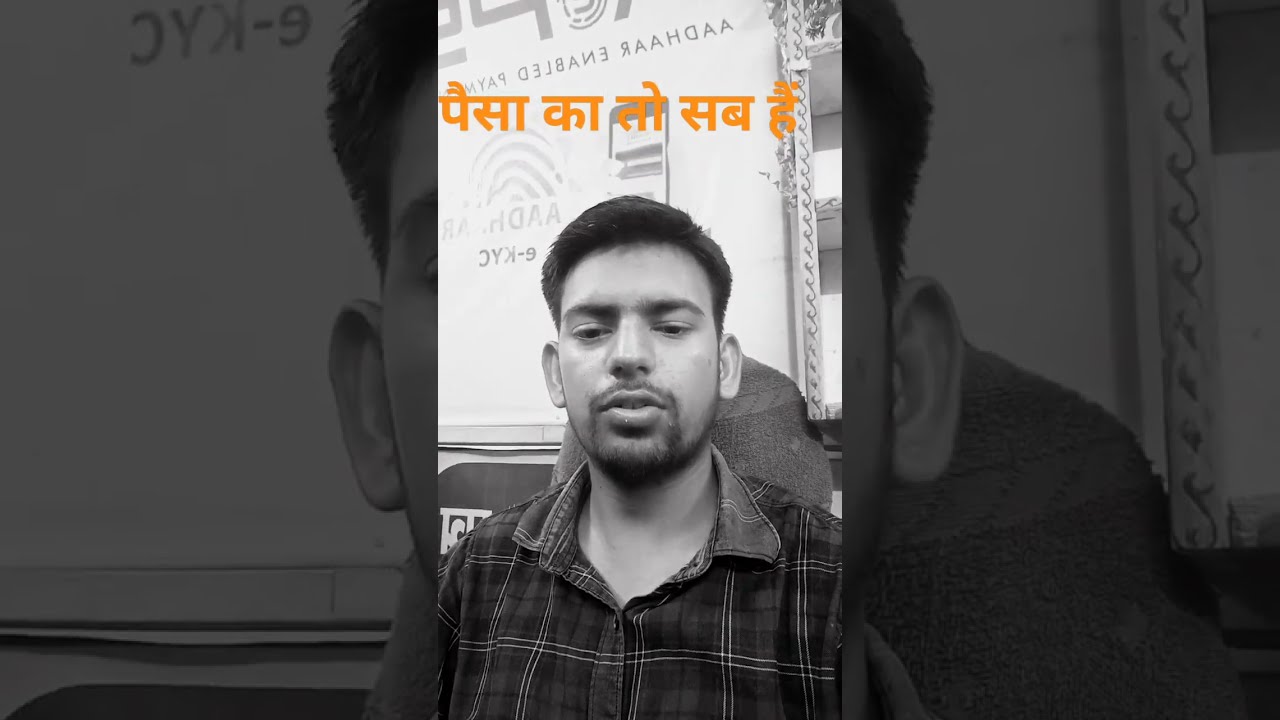The image features a young Indian man with short dark hair and a goatee, seated in a chair and wearing a plaid, long-sleeve button-up shirt with the top two buttons unbuttoned. The photograph is in black and white and shows a vertical composition with the man centered more toward the bottom half. His expression includes slightly squinted eyes and a partially open mouth, and he has distinctive large ears. There is an orange foreign script above his head, likely in an Indian or Thai language. The backdrop consists of a large banner displaying a zoomed-in, grayscale version of his face. Additional text in gray, which includes the words "ADAR enabled" and "PYAM colors," can be partially seen. The setting appears to be near a window, with no other people present in the image.